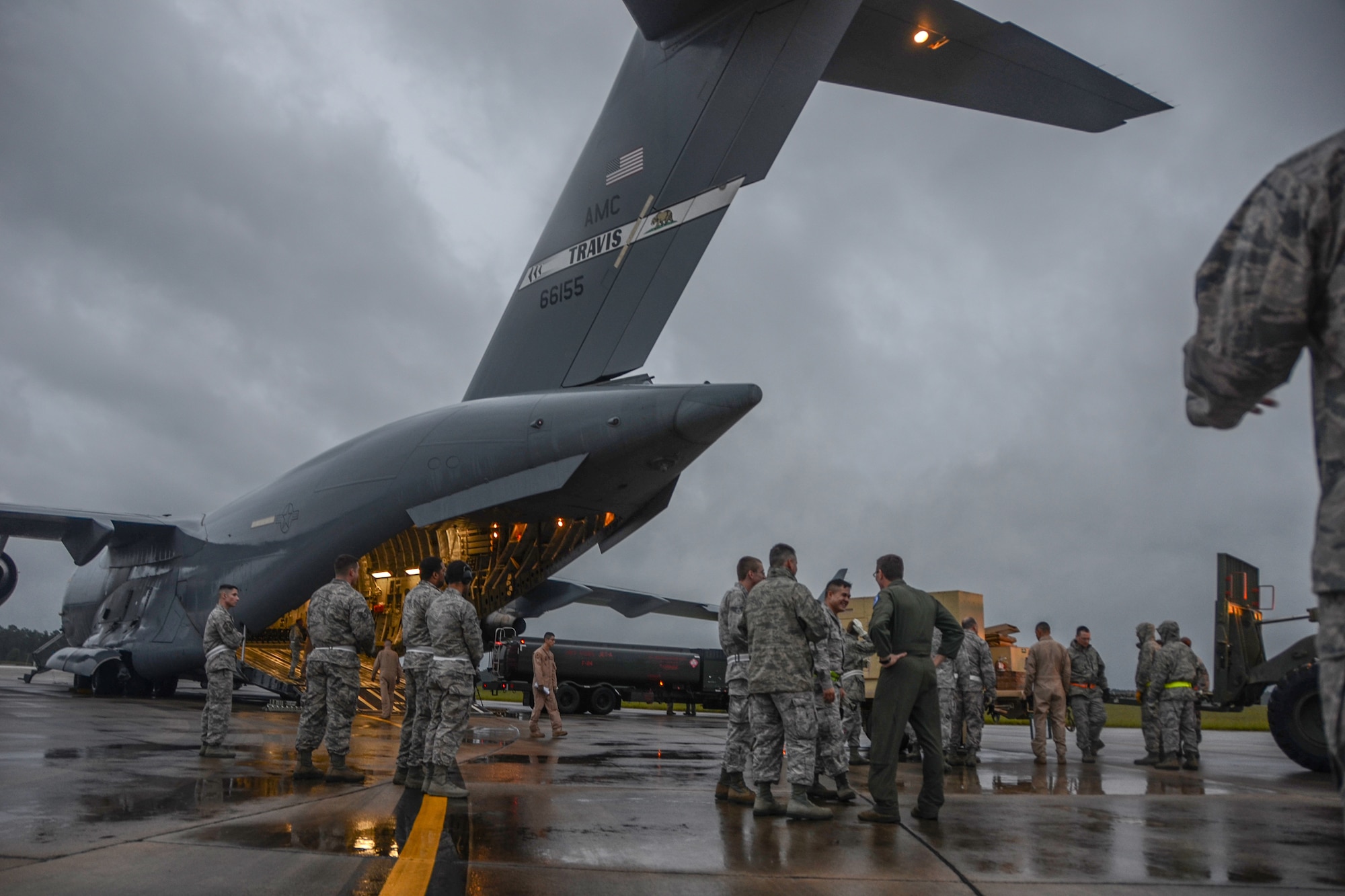The image depicts a group of approximately 15 to 20 military personnel, primarily men, wearing camouflage uniforms, congregated in a military setting. Among them, higher-ranking individuals can be identified by their distinct attire, such as a man in a dark green uniform standing toward the middle with his hand on his waist. The scene is set on a wet, rain-soaked tarmac beneath a heavily overcast, gray sky, suggesting imminent rainfall. The focal point of the background is a large, gray military aircraft positioned on the left side, bearing the United States flag, the name "AMC Travis," and the number "66155" on its tail. The atmosphere is a mix of activity, with some personnel standing around and others boarding the massive plane. To the right, a field is visible, adding to the expansive and strategic nature of the environment. The overall ambiance conveys a sense of readiness and anticipation amidst a somber, cloudy backdrop.